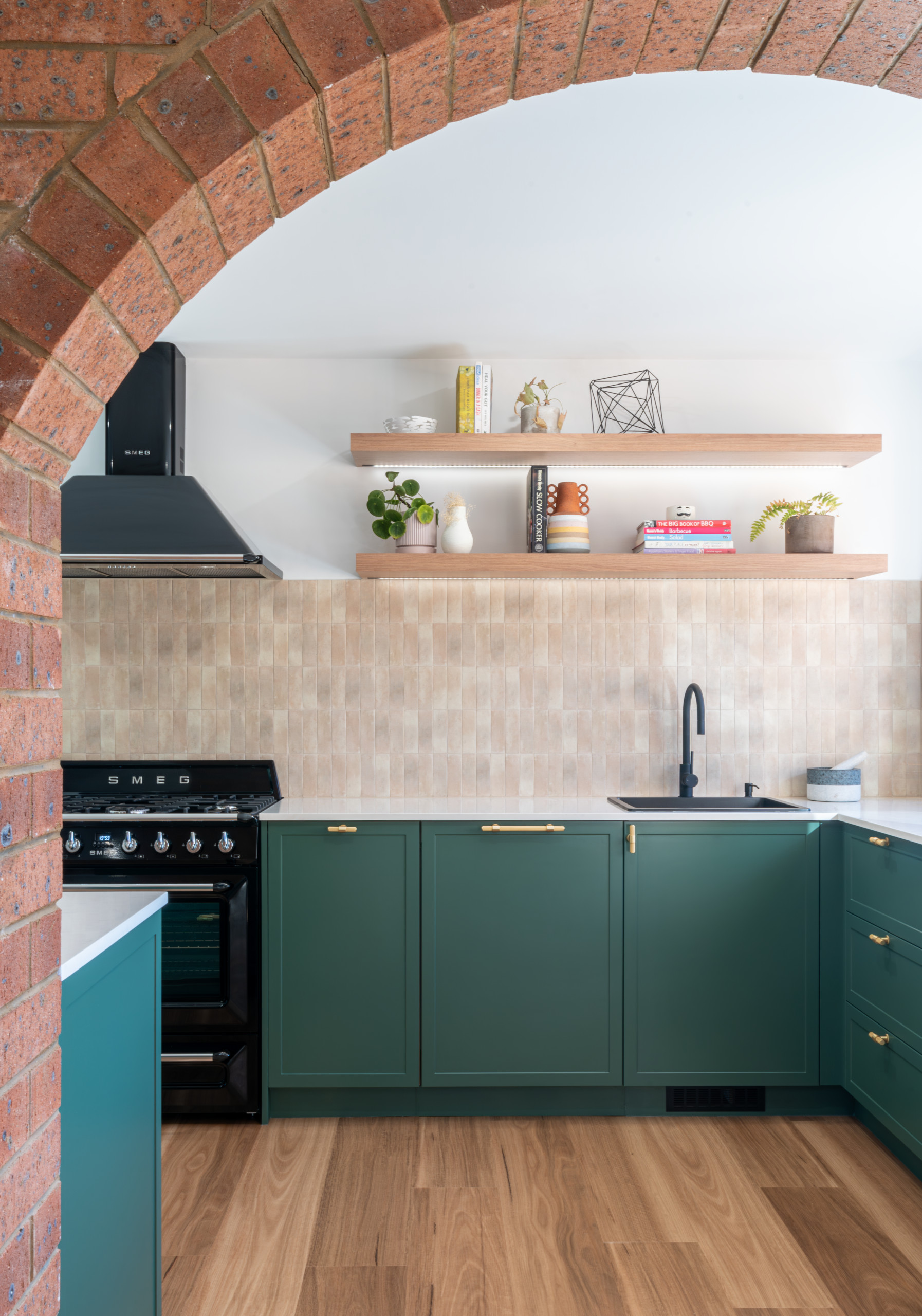This detailed photograph captures the view of a modern kitchen from an adjacent room, framed by a red brick archway. The kitchen features a wooden plank floor and green L-shaped cabinets with gold handles, extending horizontally along the right side of the image and across the back wall. The cabinets are topped with white granite counters. A black matte sink with a black faucet is integrated into the counter. To the left, there is a black stove with silver knobs, accompanied by an exhaust hood above. The backsplash is decorated with gold tiles, contrasting with the white walls that extend above it. Two wooden shelves are installed on the white wall above the backsplash, holding potted plants, books, and a cat statue. The overall color palette includes black, brown, green, gold, and white, lending the kitchen a cohesive and modern aesthetic.